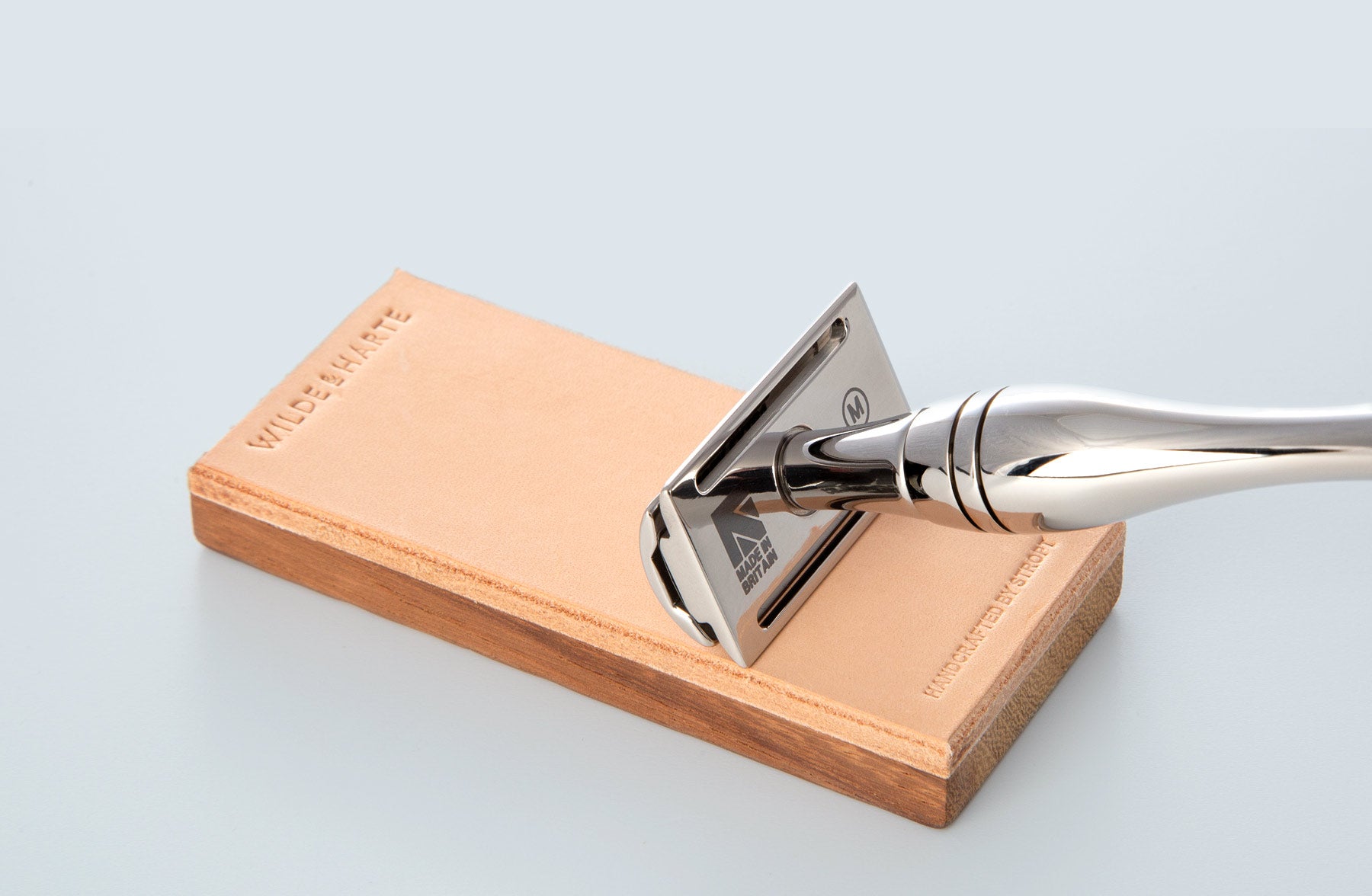The image features a sleek, silver straight-edge razor with a reflective chrome finish, lying horizontally on a rectangular pen holder. The handle of the razor, which has "Made in Britain" stamped on it, features two black rings and a distinctive bulge in the middle. The pen holder itself consists of a medium wood base topped with a light tan leather surface that spans its entire length. The leather is embossed with the text "Wilde Harte" at the top. Beneath the text on the leather, you see the silver razor, giving the impression of being sharpened or displayed for its sharpness. The scene is set against a clean, light gray background, enhancing the product's professional and polished look. The overall image appears to be a high-quality photograph or an extremely realistic illustration, showcasing the intricate details of both the razor and the pen holder.